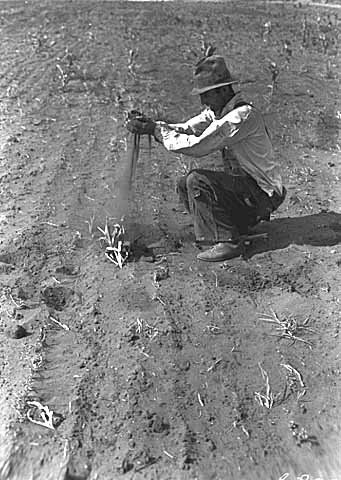This black and white photograph captures a poignant scene likely from the Dust Bowl era, depicting a forlorn farmer in a barren field. The man, squatting with his feet on the ground and body hovering just above, is clothed in a long-sleeved white shirt and dark pants, possibly overalls. He wears a brimmed hat, either a fedora or a bucket shape, to shield his face from the harsh elements. Pointed and rugged work boots adorn his feet. Delicately, he holds dirt in his hands, allowing it to sift through his fingers over the dried, sparse vegetation at his feet, which appears withered and poorly grown, with visible but barren rows of planted crops stretching into the desolate landscape. The farmer's expression conveys a sense of loss as he assesses the failed crops around him, underlying the grim reality of the agricultural devastation of the period.